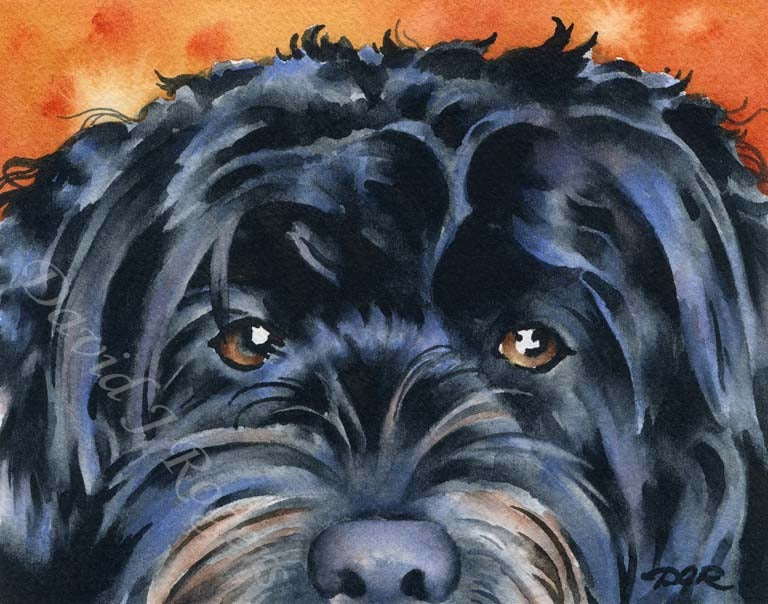This detailed painting captures the intense gaze of a black dog with dark brown eyes, set against a dynamic orange and white background with painted splooges. The artwork, focusing predominantly on the dog's face, extends from just below the nose to the top of the head, with the snout partially obscured. The textured fur, depicted in strokes of black, gray, with tinges of blue, and lighter patches of brown and white near the nose, conveys a sense of depth and realism. The dog's ears are mostly hidden, emphasizing the facial expression, particularly the eyes. A watermark diagonally across the painting reads "David J. Rogers," with a signature, "DGR," in the lower right corner, confirming the artist's identity.